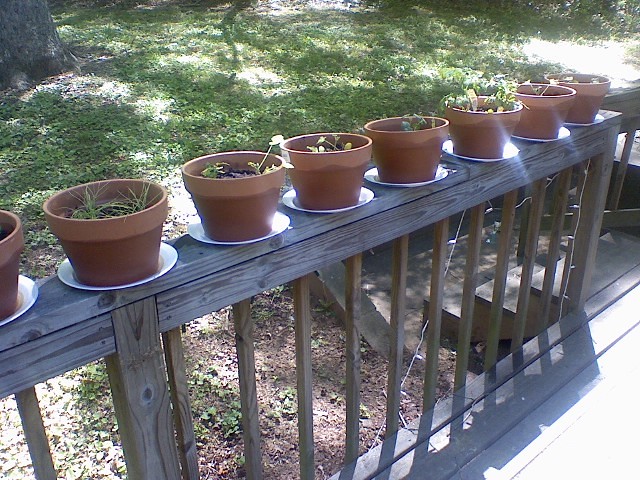This image depicts eight ceramic flower pots, each resting on white plates, arrayed along the top of a wooden railing that forms part of a porch. The railing, made of light brown wood with spindles, connects to stairs leading down to a grassy area. The vibrant green grass and part of a tree root are visible in the background. The flower pots are varied in color, including light and dark brown, and contain different plants: one with a grassy structure, another with a leaf, a third with a yellow leaf, a fourth with greenery, and a fifth with a larger plant. The details of the sixth and seventh pots are less distinguishable due to the sunlight. This scene gives a charming view of a garden setup on someone's deck.